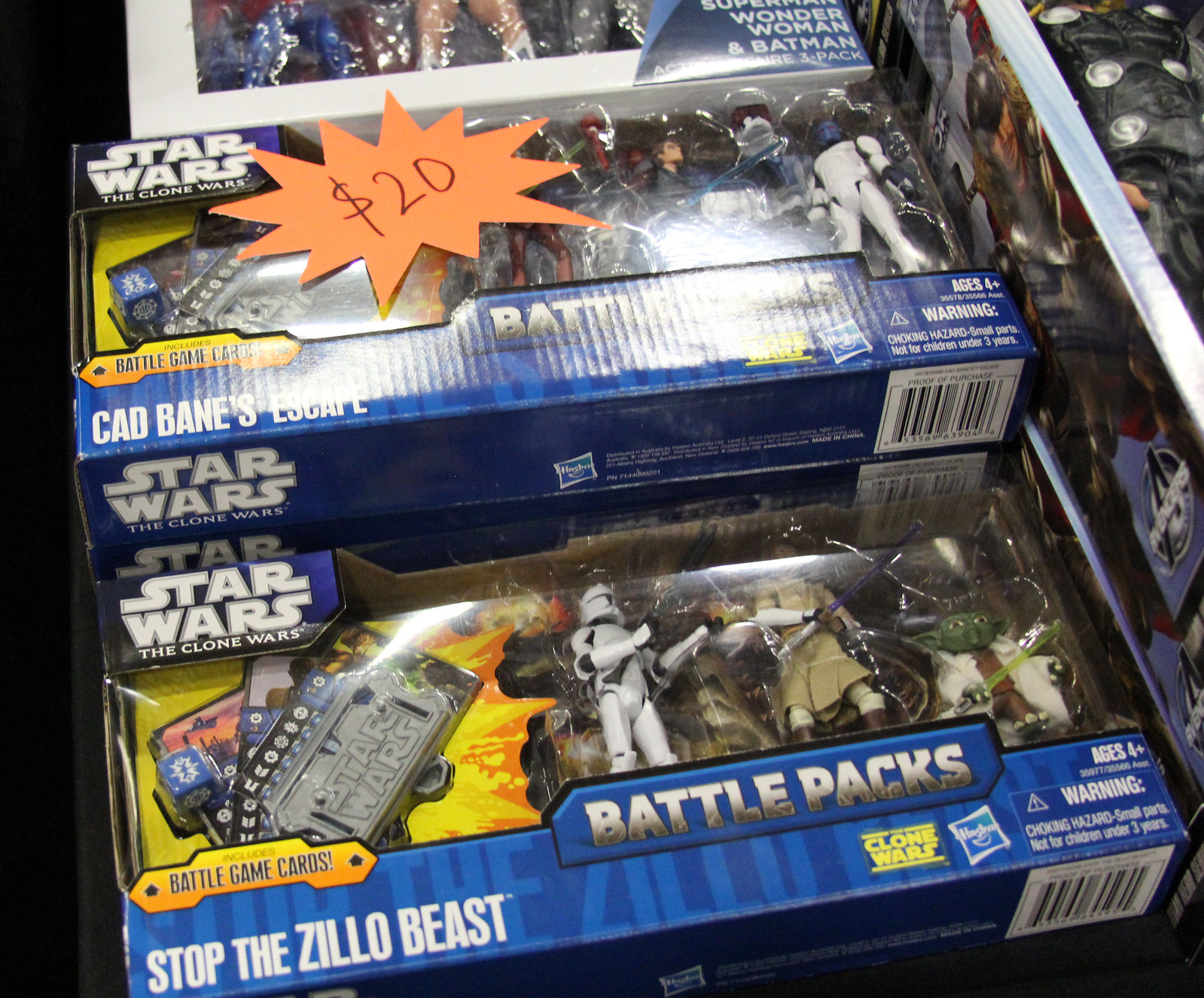This is a detailed color photograph showcasing a stacked display of boxed Star Wars action figure sets, likely from the Clone Wars series, potentially in a store setting. The boxes are blue with clear plastic windows revealing the figures inside. The box at the bottom, prominently labeled "Stop the Zillow Beast," contains several action figures including Stormtroopers, Yoda, and another Jedi with lightsabers, and features battle game cards. Another box higher up, titled "Cad Bane's Escape," also contains multiple action figures and has an orange star-shaped handwritten label marked $20. The collection evokes a nostalgic feel, possibly from the 80s-90s era, and is meticulously arranged for sale.